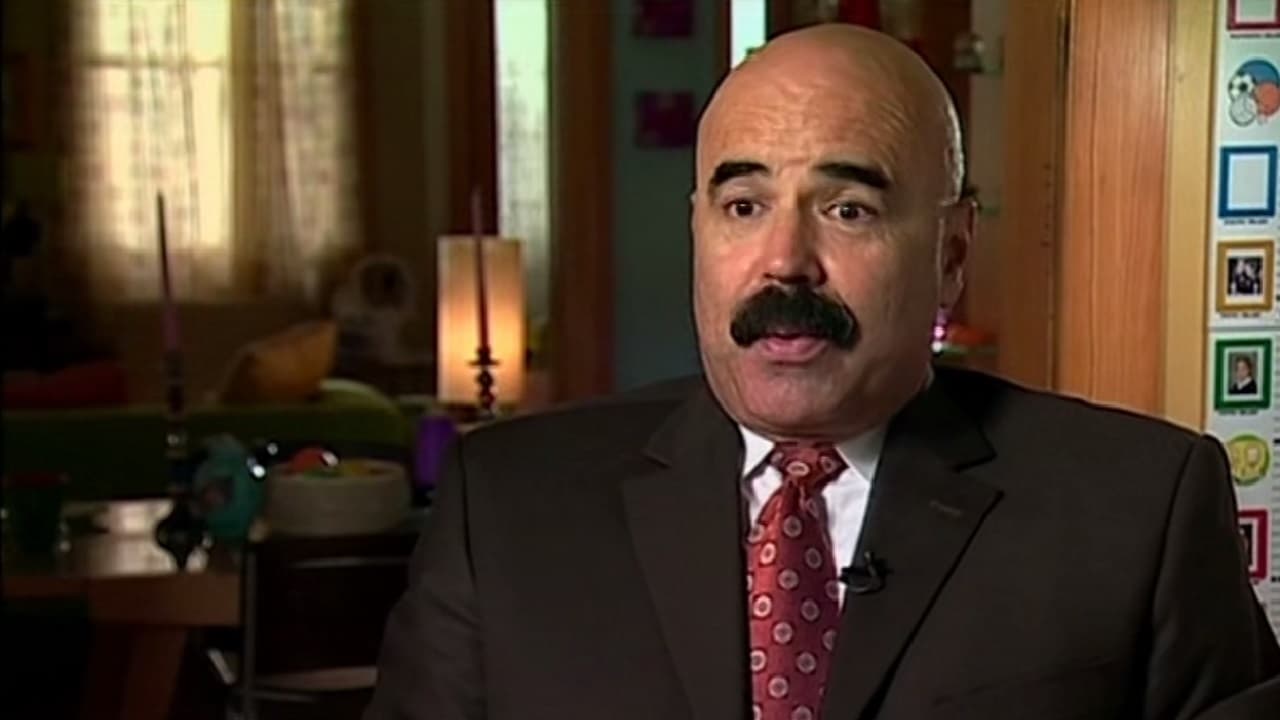The image depicts a bald-headed, older gentleman wearing a dark suit coat, a white shirt, and a red tie adorned with gold circles. He has thick, black eyebrows, a bushy dark mustache, and his lips are slightly pursed. The man, who appears to be participating in a TV news report due to a microphone clipped to his lapel, sits slightly off-center to the right, looking just to the left of the camera. Behind him is a room that might be part of a home or a set designed to resemble one. The background features a wooden doorway, several small framed pictures hanging on the wall, and more subdued background items including a green sofa and a wooden table with chairs. To the left, there are curtains over a window, with light filtering through them, and two candlesticks with long candles. A round, short lamp is also visible along with various other indistinct objects. The scene is lit with artificial light, with hints of natural light, contributing to an array of colors—flesh tones, blacks, reds, tans, greens, golds, and yellowish curtains.